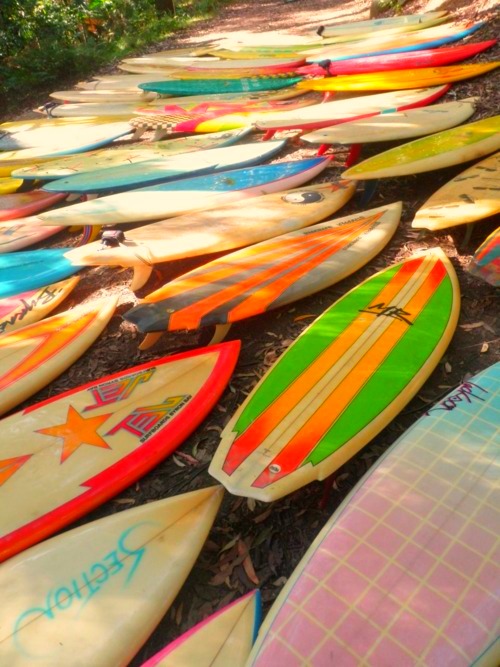This vibrant and picturesque image portrays an outdoor scene on a bright summer day, featuring an impressive collection of approximately 50 surfboards laid out on what appears to be a road or footpath adjacent to a forest. The surfboards span from the bottom to the top of the picture, creating an almost endless, visually stunning array of color and design.

The surfboards present a dazzling palette, including lime green, orange, yellow, checkered pink and blue, fluorescent greens, and reds. Some surfboards sport unique patterns and markings such as fish designs with eyes, stars, and writing. Notably, there are checkerboard patterns in purple, light blue, and dark blue, as well as boards labeled "MR" in black and "section" in bright blue lettering. A bright aquamarine blue surfboard and another in bright pink and yellow catch the eye in the background.

The surfboards lie flat on the soil, surrounded by dried leaves and a bit of shrubbery, with a few trees visible in the distance. This colorful and eclectic assortment of surfboards against the natural backdrop creates a beautiful, lively scene that's rich in detail and visual appeal.